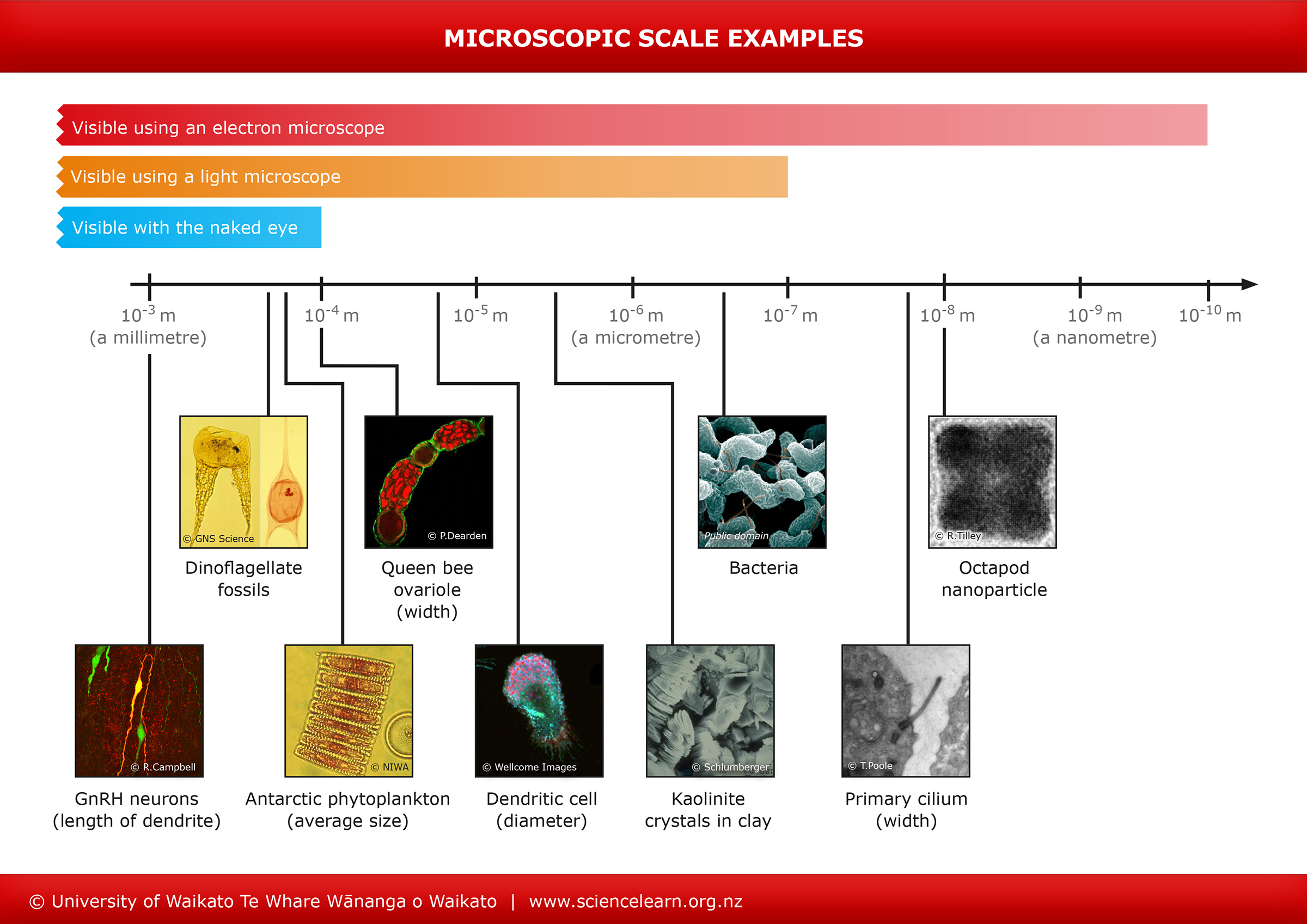This scientific graphic titled "Microscopic Scale Examples" is divided into three sections based on the visibility of items: "visible using an electron microscope," "visible using a light microscope," and "visible with the naked eye." The diagram illustrates nine different items across these scales, highlighting how each can be observed. From left to right, the smallest observable item is an octopod nanoparticle, followed by the primary cilium, bacteria, kaolinite crystals in clay, a dendritic cell, queen bee ovariole, Antarctic phytoplankton, dinoflagellate fossils, and a GnRH neuron. The items range in visibility, with fewer items visible to the naked eye and more requiring various types of microscopes. The top section contains electron microscope images, including the cilium and kaolinite crystals, while the light microscope section features images like the dendritic cell. The naked-eye section includes larger items like the queen bee ovariole. The graphic is rich in color and detail, displaying images such as a blue and purple jellyfish-like dendritic cell and light blue bacteria, all laid out for comparison. The source of the graphic is the University of Waikato Te Ware Wananga o Waikato of New Zealand, as indicated at the bottom.